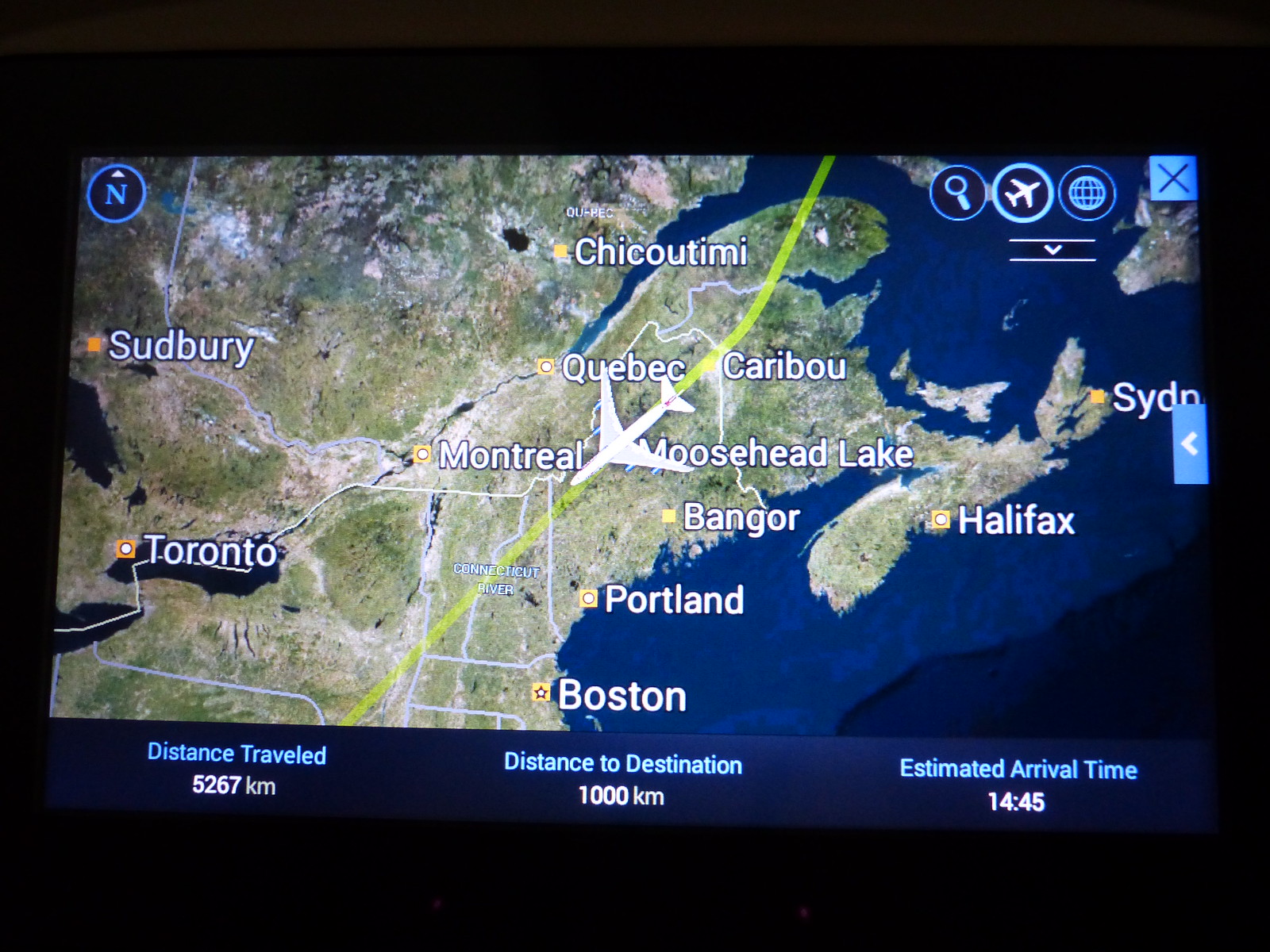The horizontal rectangular image is a detailed map, possibly a screenshot, reflecting the flight path of an airplane. The map is displayed either on a computer screen or a cell phone screen. The land is depicted in a brownish or greenish tone, while the water ranges from blue to very dark blue, especially in the lower right corner. Cities from both Canada and the United States are marked on the map. Key locations include Toronto on the far right, Sudbury, Montreal, and Quebec. 

There's also an airplane symbol approximately halfway along a yellow diagonal track that runs from Canada down through the United States, with major American cities like Portland and Boston marked towards the bottom of the map. The map provides various symbols, including a magnifying glass and a globe symbol to the right, along with a capital 'N' inside a circle in the upper left indicating north. 

Words in a mix of upper and lowercase letters identify cities such as Chicoutimi at the top center, Caribou, Bangor, and Halifax near a peninsula. Further annotations include Head Lake and Cedo on the far right, near the coastline. Additionally, a banner at the bottom displays important flight information: "Distance traveled: 5267 kilometers, Distance to destination: 1,000 kilometers, Estimated arrival time: 1445." This text is shown in blue on a blue banner, with a black banner beneath it.